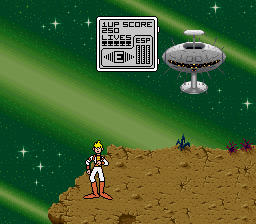This is a square, color photograph showcasing a scene from an arcade-style video game. The background is a textured green sky with alternating light and dark diagonal green stripes, interspersed with white stars. Dominating the top right corner is a silver, disc-shaped spaceship with yellow and red lights around its circumference. To the left of the spaceship, a silver control panel with some buttons displays text indicating "1 UP", "250 LIVES," and "ESP", though it's somewhat too small to be completely clear. 

At the bottom of the image, there is a rough, cratered terrain of tan color, scattered with small rocks and cracks, and dotted with red and blue plants. In the center of this landmass stands a small human character with short blonde hair and fair skin, wearing a decorative white top and shorts that reach the knees. The character's outfit includes blocks of color in black and yellow, and they are sporting high, orange-colored boots. The character is positioned as if facing the observer, giving a sense of anticipation and engagement in this vibrant, galactic setting.